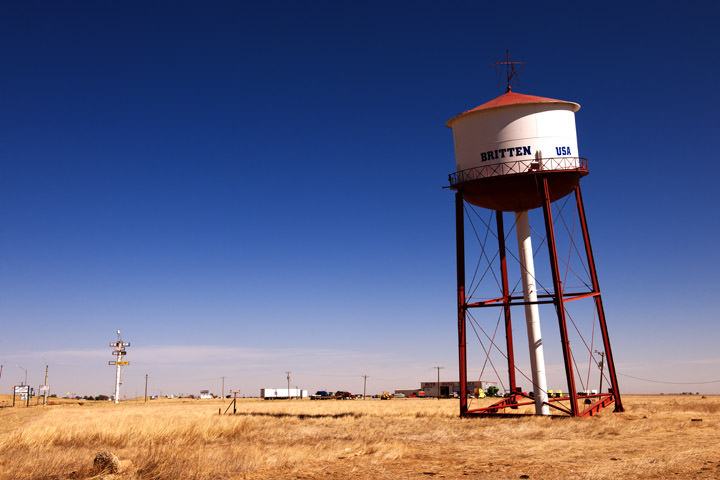In the foreground of this outdoor scene, a precariously tilting water tower stands, leaning to the left. Positioned slightly to the right side of the image, the water tower is elevated on rust-colored red legs that support two sections leading up to the water tank itself. The tank is white and topped with a red, cone-shaped roof. Bold blue letters on the tank spell out "Britain, USA." 

Underneath the tank, a white pipe extends from top to bottom, interspersed with stabilizing wires and zigzags. Notably, one foot of the tower has dug deep into the dry, yellow-brown grass, causing the opposite foot to lift off the ground. Surrounding the base, a safety barrier is visible alongside a bolt that secures the structure.

In the background, a highway populated with vehicles, including a white 18-wheeler truck, stretches across the middle of the image. To the left, a white post sign with multi-colored directions stands, although the text is too distant to read. Further back, a power line runs parallel to the road. 

The sky above is a vivid and gradient blue, darkening towards the top and lightening with haze near the horizon. A few scattered clouds float at the bottom of the sky. Behind the highway, structures including what might be a trailer and a low-story wooden building hint at a once-active, now seemingly abandoned area. The arid, unkempt ground and the leaning water tower imply a sense of desertion and time passed.